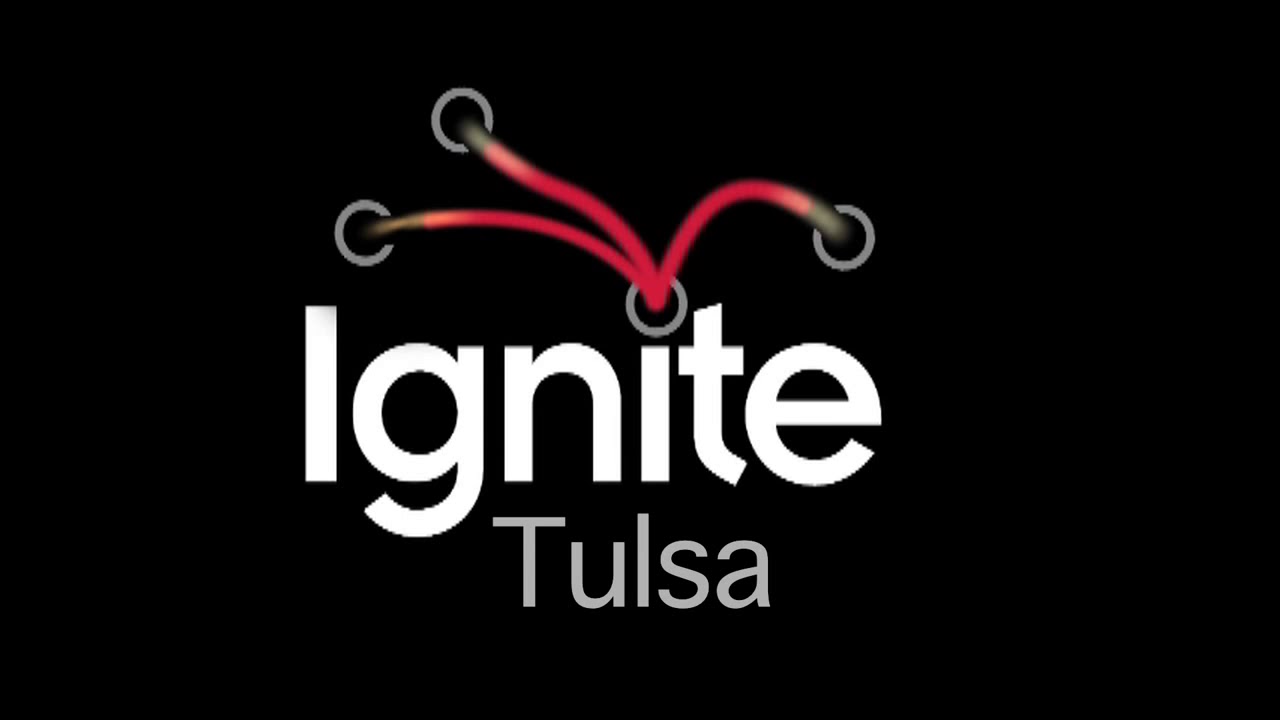The image is a sleek advertisement set against a solid dark black background. Central to the image is the word "Ignite" in large, clean, white letters with a capital 'I' and the rest in lowercase. Directly beneath it, in a smaller, light gray font, is the word "Tulsa," with a capital 'T' and the other letters in lowercase. Above the word "Ignite," four gray, hollow circles are arranged on the wall. The central circle has three red wires stemming from it, transitioning to black at their ends. Each wire extends towards and terminates in one of the other hollow circles: two wires go towards the left, with one curving slightly upward and the other extending almost horizontally, while the third wire loops upward in an upside-down U-shape towards the right. The overall layout is clean, with a modern and minimalistic design.